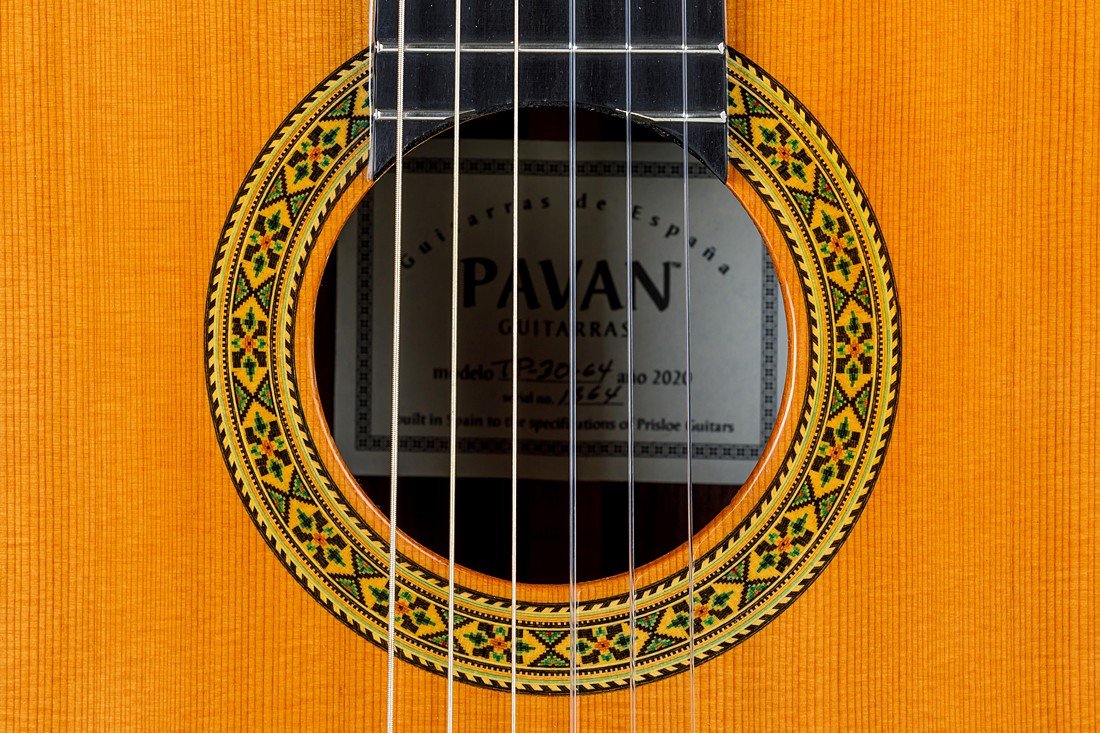This close-up, horizontal photograph showcases the central portion of an acoustic guitar's body. The surface of the guitar is made of light brown wood, adorned with intricate designs circling the central sound hole. These designs feature a combination of black, green, and red colors, creating a decorative border. Running vertically across the image are the guitar's six silver strings, extending from the top to the bottom of the frame. At the top of the sound hole, a black section with white horizontal lines, part of the neck's end, intersects the design. Inside the circular hole, a white rectangular sticker is visible. The sticker contains black writing, prominently displaying "Pavan Guitares," followed by additional text including model numbers and serial numbers.